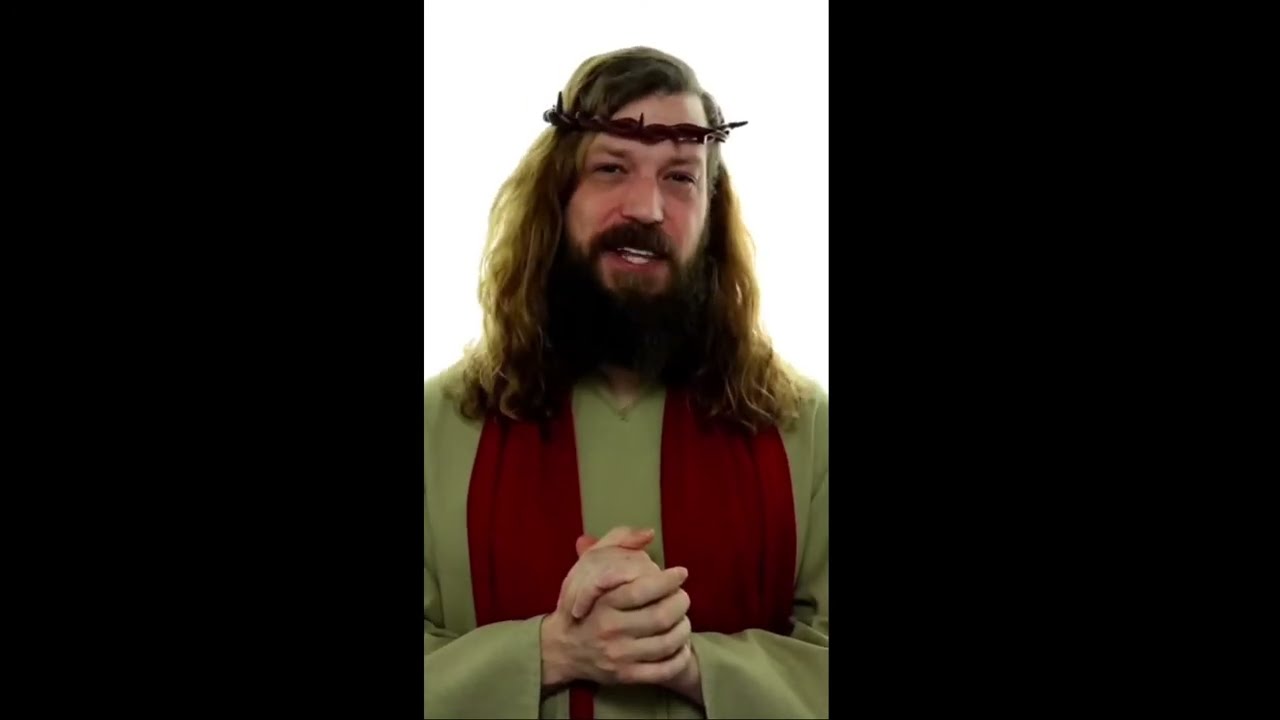The image features a man who appears to be impersonating Jesus Christ. He has light brown, wavy hair that falls just below his shoulders and a prominent, bushy brown beard and mustache. His skin tone is pale with a reddish hue, and he has circles under his eyes. He wears a brown braided leather headband across his forehead. A crown of thorns with visible spikes sits atop his head. Dressed in a long-sleeved, dark beige or tan robe with a v-neck, he also has a red stole draped around his neck, extending down on either side of his chest. The man's hands are clasped together in front of him, and his mouth is slightly open, showing his upper and lower teeth. The image has a bright white background behind the man’s head and shoulders, bordered by thick black rectangles on the left and right sides, making the central photo appear narrow. The man is looking directly at the camera, emphasizing his intent to mimic the likeness of Jesus Christ.